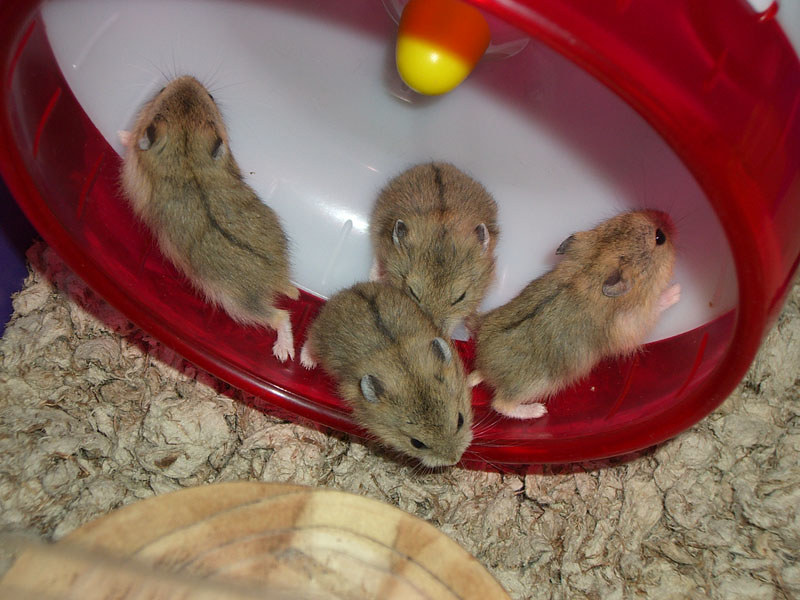The photograph captures a close-up view of four light brown hamsters with distinct black stripes running down their backs, inside their cage. The bottom of the cage is covered with beige wood shavings, providing a soft, natural base. Central to the image is a red and white hamster wheel, with a transparent red outer ring and a white inner section. A small yellow ball is attached to the side of the wheel. All four hamsters are engaging with the wheel, either slowly running or pushing against each other. Their small ears and pink feet add to their endearing appearance, emphasizing their delicate features. To the side of the wheel, a small wooden structure, possibly a tower, can be seen amidst the gravelly-looking floor of the cage. The overall scene is lively and detailed, capturing the playful nature of these little creatures in their habitat.